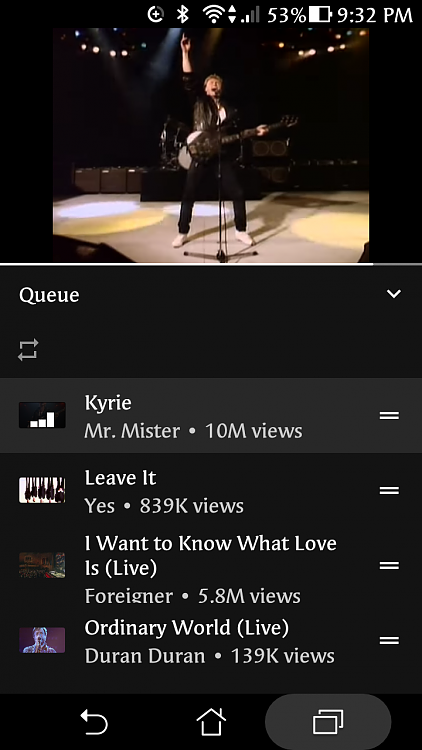This detailed caption describes an image that appears to be a screenshot taken from a smartphone. At the very top of the screen are several status icons including Wi-Fi, Bluetooth, signal strength, and battery level, indicating the time as 9:32 PM. The background of the image is predominantly black. The upper third of the image features a white man, seemingly on stage, dressed in all black except for his white tennis shoes. He appears to be singing while playing a guitar. The stage is brightly lit with white, yellow, and beige lights, with additional illumination from lights on either side of him. 

Beneath the stage scene is the word "Q," referencing a list of songs available to choose from a website. The song titles and their view counts are as follows: 
1. "Curie" by Mr. Mister with 10 million views.
2. "Leave It" by Yes with 839,000 views.
3. "I Want to Know What Love Is" (Live) by Foreigner with 5.8 million views.
4. "Ordinary World" (Live) by Duran Duran with 139,000 views.

At the bottom of the screen are three icons: a reverse arrow for going back, a home button, and what appears to be a split screen icon.